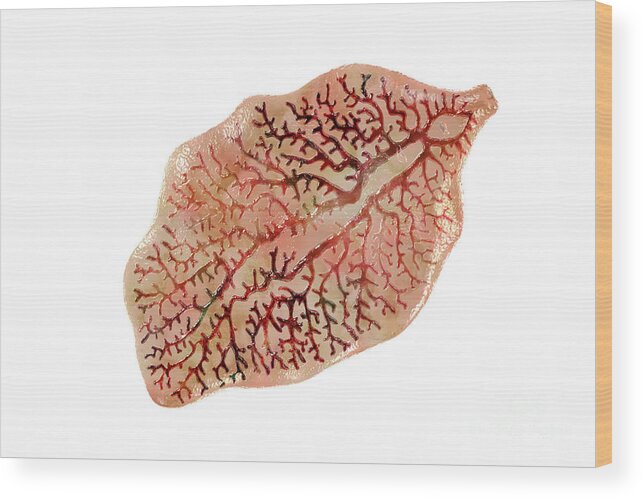The image features a piece of artwork presented in a landscape-oriented rectangular frame made of wood. The front face of the wood is painted white, while the edges are in their natural wood color, about an inch thick. The artwork itself depicts a leaf, diagonally positioned with the tip pointing towards the lower left and the stem extending to the upper right. The leaf is predominantly a pinkish-brown or flesh color with a slightly shiny finish. Its edges are wavy and scalloped, contributing to an organic look. The interior of the leaf is detailed with intricate, dark reddish-brown veins that branch out extensively, resembling a network of rivers. The entire image has no text, focusing solely on the artistic portrayal of the leaf against the white background.